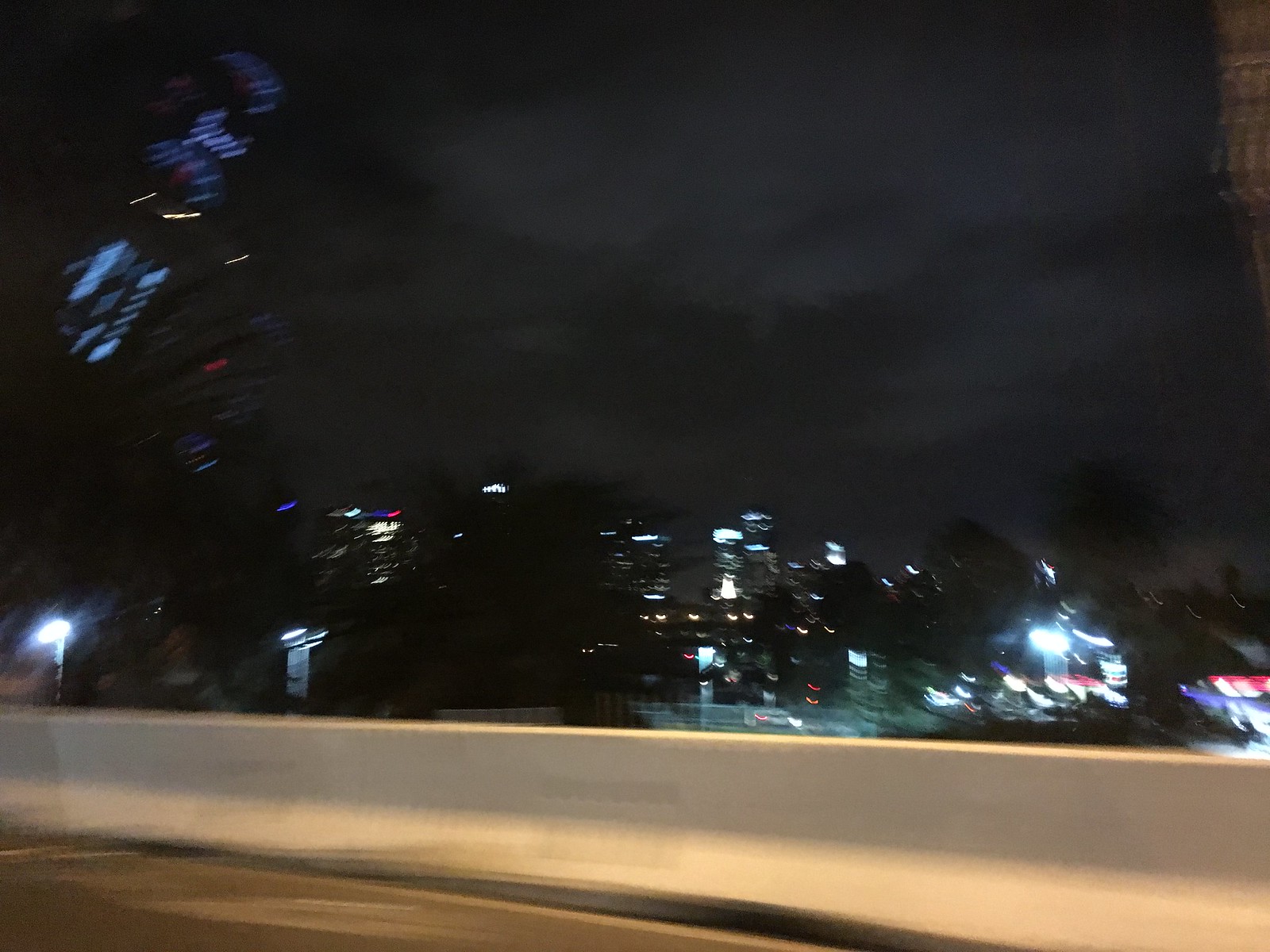This photograph, taken at night from inside a car, captures a panoramic view of a city's illuminated skyline. The vantage point appears to be from a highway or elevated road, characterized by a prominent white concrete barrier in the foreground. Beyond the barrier, the cityscape unfolds with numerous skyscrapers and buildings, their lights glowing vibrantly. The scene is slightly blurred, giving a dreamy quality to the image, and reflections from the car's window create a ghostly overlay of the city lights and skyline. Dark trees emerge as silhouettes against the brilliantly lit buildings. Above, the night sky is partially shrouded by grayish clouds, adding to the atmospheric depth of the photograph. The overall impression is one of urban splendor viewed through a transient moment on the move.